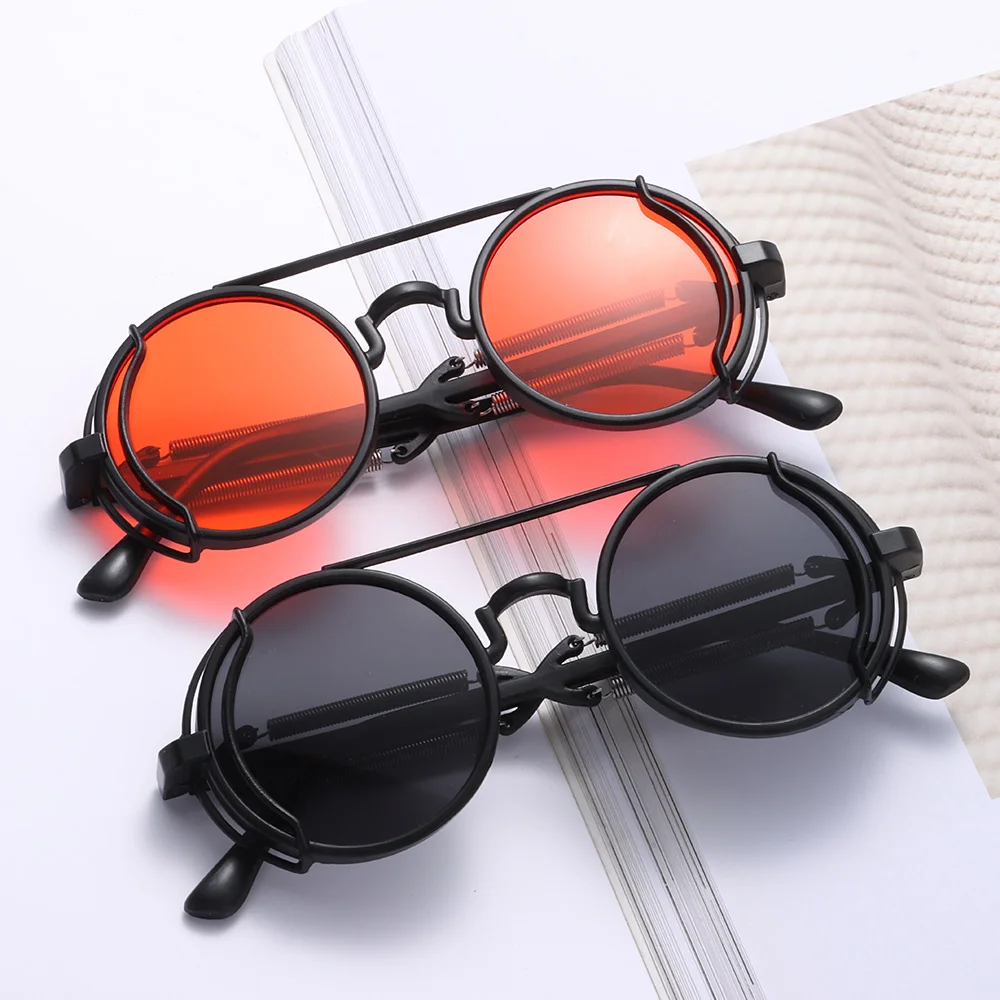The image features two pairs of sunglasses resting on a white surface. Both pairs share the same unique design but differ in their lens colors. The top pair has circular, reddish-orange lenses, reminiscent of rose-colored glasses, while the bottom pair sports solid black lenses. Each pair is crafted with black plastic rims and has notable metal springs on the arms, two on each side, making them more flexible and durable. The springs are silver and the arms of both sunglasses are black plastic, extending from the circular lenses. The nose pieces are distinctively shaped for a snug fit. Additionally, the white backdrop includes a textured surface, possibly resembling a paper towel, visible on the right side of the image, adding a subtle detail to the composition.